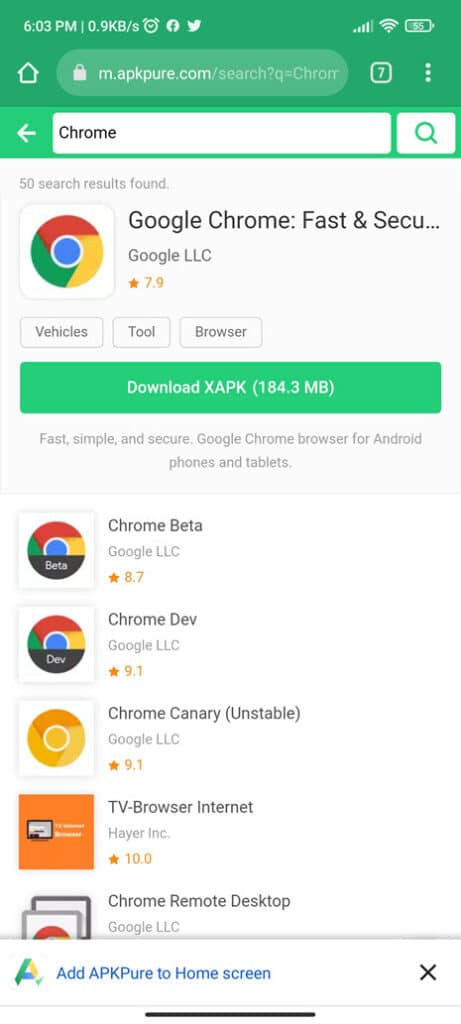The image's background is predominantly green, displaying the time as 6:03 p.m. The main focus is a webpage featuring an image of a house. At the top, within a search bar, the URL "m.apkpure.com" is visible alongside another search box containing the word "Chrome".

The page indicates that 50 search results have been found for Google Chrome, highlighted with the text "Google Chrome FASTNSECU" followed by three dots. A familiar Google logo consisting of red, yellow, green circles, and a small blue circle is present, suggesting the option to download the browser.

A prominent download button labeled "Download XAPK (184.3 MB)" is visible, offering the download of Google Chrome. Below this, ratings and details of various Chrome versions are provided: 
- Chrome Beta by Google LLC with a rating of 8.7 stars.
- Chrome Dev with a rating of 9.1 stars.
- Chrome Canary with a rating of 9.1 stars.
- TV Browser Internet with a perfect rating of 10 stars.
- Chrome Remote Desktop.

Finally, at the bottom, a search bar prompts users to "add APKPure to home screen."